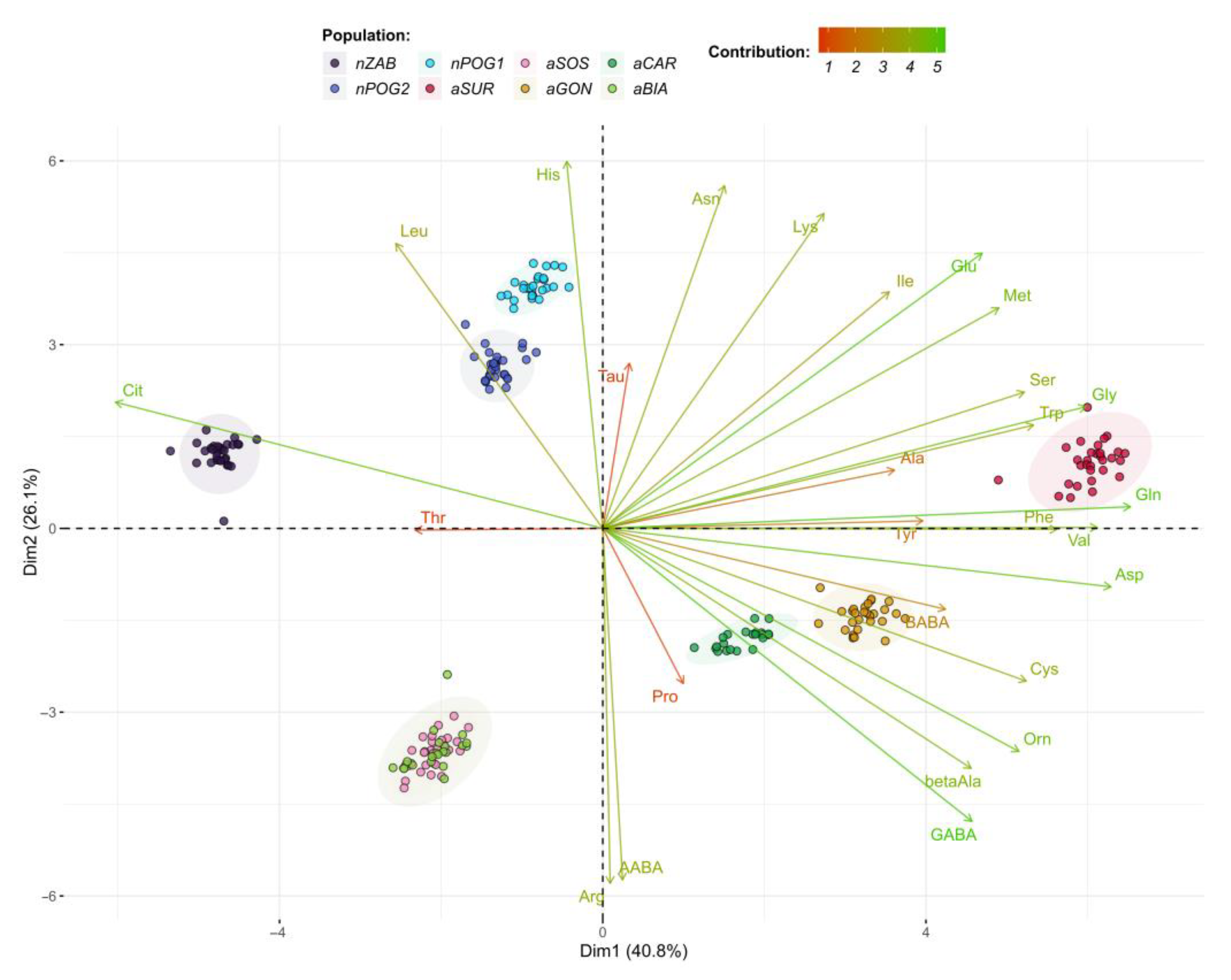The image is a graph illustrating population distribution across four quadrants, formed by intersecting vertical and horizontal axes at the origin (0,0). From the center, various arrows radiate outwards in different directions, predominantly green but interspersed with red, orange, and yellow arrows. Population data is visually represented by clusters of colored dots dispersed within each quadrant. The graph includes a legend at the top explaining that the dots signify population categories, each colored dot representing a different group: purple for nzab, sky blue for npog1, pink for asos, dark green for acar, regular blue for npog2, red for asur, orange for agon, and light green for abia. Additionally, a gradient bar ranging from red to green quantifies contribution, scaling from one to five.

Specifically, the upper left quadrant features clusters of light blue, dark blue, and purple dots. The upper right quadrant contains a single cluster of red dots situated slightly above the midline of the x-axis. In the lower left quadrant, green and pink dots are clustered together in the same region. The lower right quadrant showcases clusters of dark green and orange dots. Despite the detailed visualization, the graph lacks explicit labels for axes or a clear title, leaving the scope of the data somewhat ambiguous.